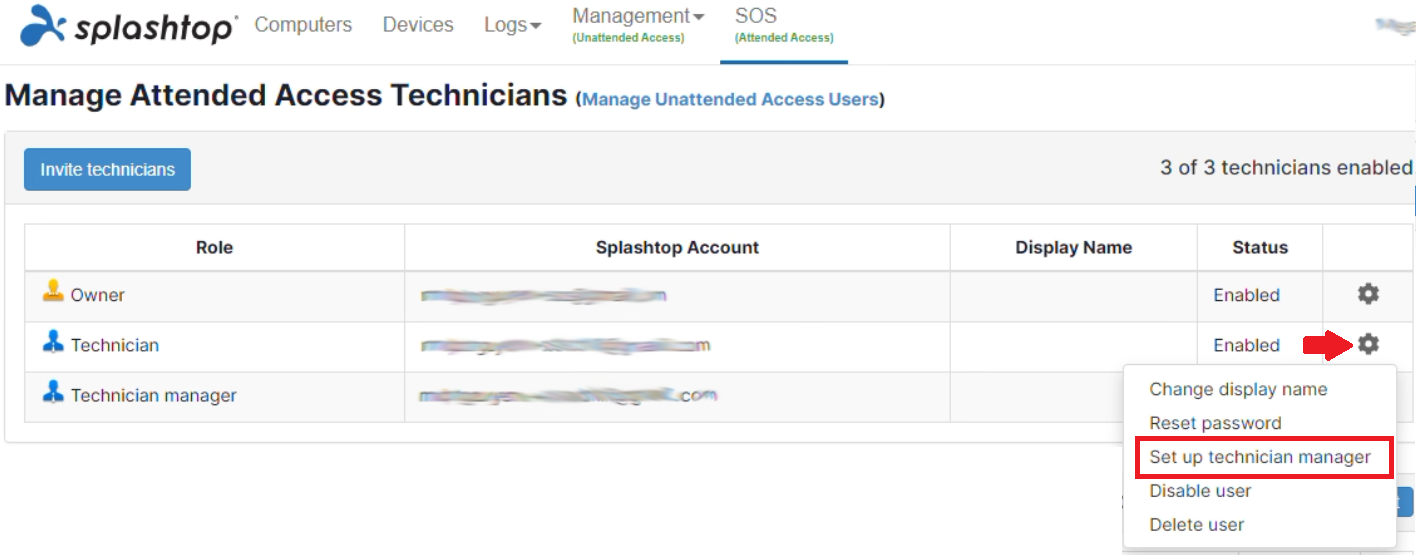The image captures a screenshot of a computer or phone displaying the Splashtop interface, which is a remote desktop software. The screen prominently features several menu options, including "Computers," "Devices," "Logs," and "Management." It displays categories such as "Unattended Access" and "Attended Access," both highlighted in green. Below these categories, there's a section titled "Manage Attended Access Technicians," with a parenthetical note that reads "Manage Unattended Access Users."

In this section, there is a clickable button labeled "Invite Technicians." Underneath, it lists different roles: "Owner," "Technician," and "Technician Manager." Each role is associated with an obscured email address, presumably for privacy reasons, where the text has been smudged out. 

Further down, the status for each technician is indicated as "Enabled." Additional options are available in a dropdown menu, including "Change Display Name," "Reset Password," "Setup Technician Manager," "Disable User," and "Delete User." The "Setup Technician Manager" option is highlighted with a red rectangle, and a red arrow points directly to this selection, drawing attention to it. The interface shows that three out of three technicians are currently enabled.